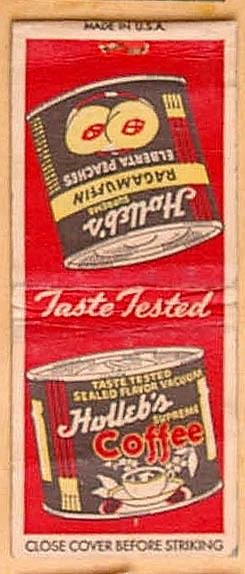This is a detailed image of a vintage advertisement for Holub's canned peaches and coffee, seemingly framed. The ad prominently features two Holub's coffee cans, one positioned upside down atop the other, and both sporting a distinctive color palette of black, yellow, and red. The advertisement, set against a red background with white accents, is captioned with "Made in the USA" at the top, and "Close cover before striking" at the bottom. Between the cans, the ad highlights "taste tested" and "sealed flavor vacuum." The top can displays an image of a peach sliced in half, while the bottom can depicts a coffee cup on a saucer, filled with steaming coffee. Holub's brand name appears in vintage font on the cans, with 'Holub's' in white and 'Coffee' in red. This nostalgic image encapsulates the essence of mid-century product marketing.